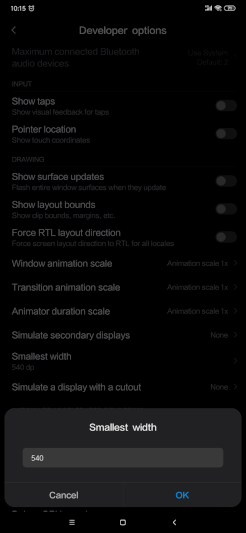The image features a dark black background, which gives the impression of a somewhat obscured view due to a pervasive gray tint, making the elements on the screen blend together in a blur. At the top of the screen, there is a header labeled "Developer Options." Below the header, a list of settings is visible, which includes options such as "Show taps," "Pointer location," "Show surface updates," "Show layout bounds," "Force RTL layout direction," "Window animation scale," "Transition animation scale," and "Animator duration scale." Additionally, there is an option to "Simulate secondary displays" and another label that partially reads "Simulate a something with the cutout." 

Towards the bottom, there is an editable field labeled "Smallest width," which currently displays the value "540." This section is enclosed within a box. Just below this field, on the left side, there is a button labeled "Cancel" and, on the right side, a blue button labeled "OK." The overall appearance is typical of a settings menu in a developer or advanced configuration mode on a device, where various advanced customization options are available.